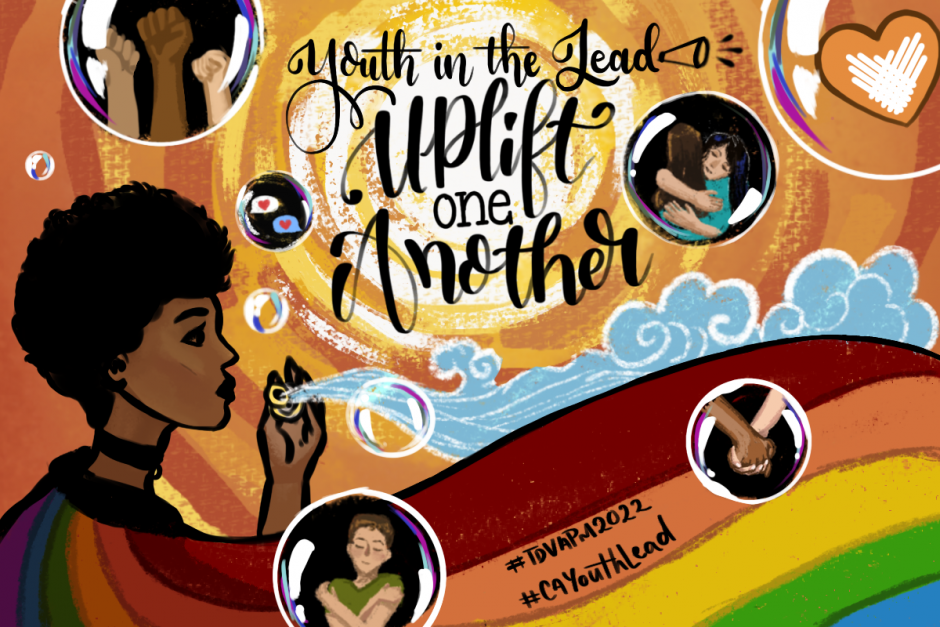The image is an illustrated advertisement with a brown-yellow background, featuring a black woman in the foreground facing right. She has a pixie haircut and wears a thick black choker. She is depicted blowing bubbles using a circular gold object, and blue wind or cloud-like elements emerge from this object, flowing over her rainbow-colored cape. The cape stretches across the bottom of the image, where the hashtags "#TOVA PM 2022" and "#C4YouthLead" are prominently displayed in pink.

Various bubbles are seen floating throughout the image, each containing different scenes: 
- A bubble in the top left features three raised fists of different skin tones: one black, one lighter brown, and one Caucasian.
- Another bubble in the upper right contains two crossed hands, forming a heart shape.
- A bubble nearby shows two women hugging, both wearing blue shirts.
- Further, a bubble in the bottom middle shows a man in a green shirt hugging himself.
- One bubble depicts a white and a black person holding hands.

Prominent text in the center reads, "Youth in the Lead, Uplift One Another," accompanied by a small microphone icon, emphasizing the message of youth empowerment and solidarity.